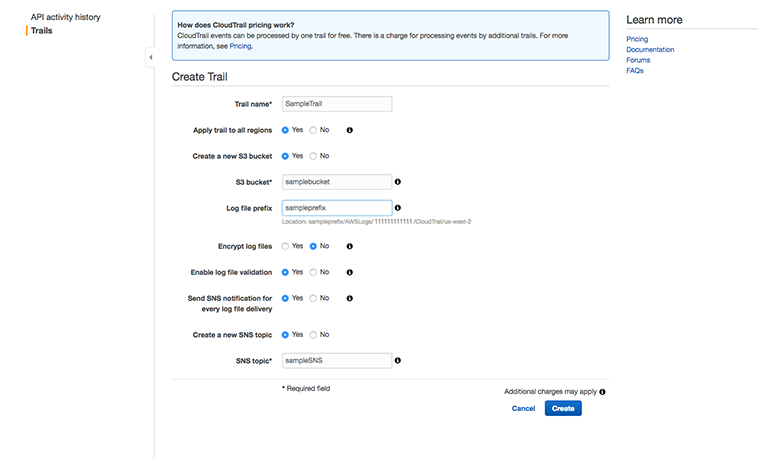The image displays the "API Activity History" page of CloudTrail, with the word "Trails" prominently located on the top left corner. To the right, a section titled "How does CloudTrail pricing work?" is visible, explaining that CloudTrail events can be processed by one trail at no cost, while additional trails incur a charge. 

The page includes a form for creating a new trail, with fields such as "Trail Name," a checkbox to "Apply trail to all regions," and an option to create a new S3 bucket. Some of the fields have asterisks indicating they are required. For each field, there are information icons providing additional guidance for users. 

On the right-hand side, there are several helpful links for users to further understand CloudTrail, including "Learn more about pricing," "Documentation," "Forums," and "FAQs." 

At the bottom of the form, there are two buttons: a blue "Create" button to submit the form and a "Cancel" button to discard the changes. The image appears to be a part of a software or programming interface related to server-side settings, likely for those managing a website or cloud services.